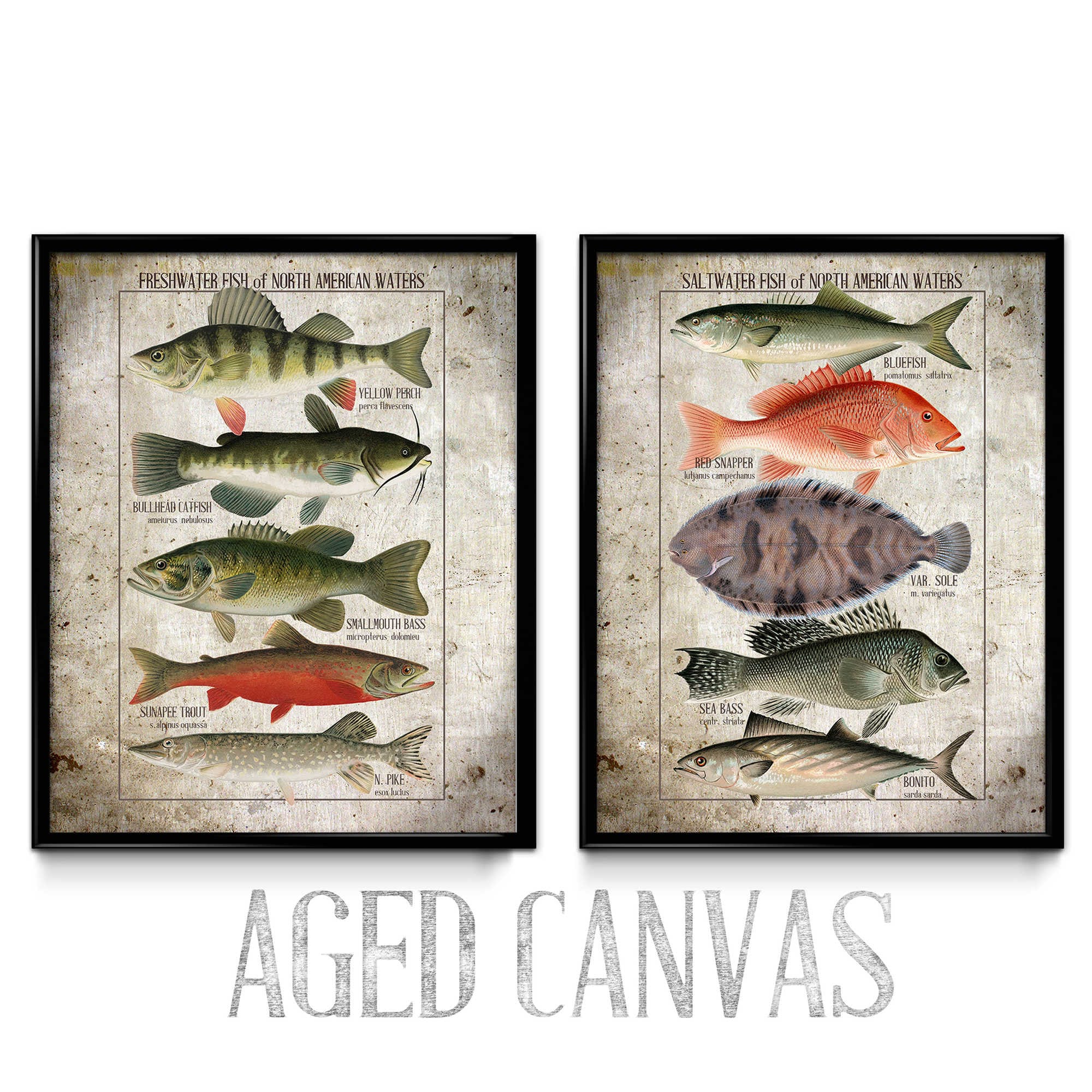The image depicts two rectangular, black-framed posters, each showcasing five meticulously drawn fish oriented horizontally in rows. The left poster is titled "Freshwater Fish of North American Waters" and features the yellow perch, bluehead catfish, smallmouth bass, sonar pea trout, and end pike. The right poster is titled "Saltwater Fish of North American Waters" and includes bluefish, red snapper, varso, sea bass, and bonito. Both posters have a gray and white background and the phrase "aged canvas" written at the bottom.